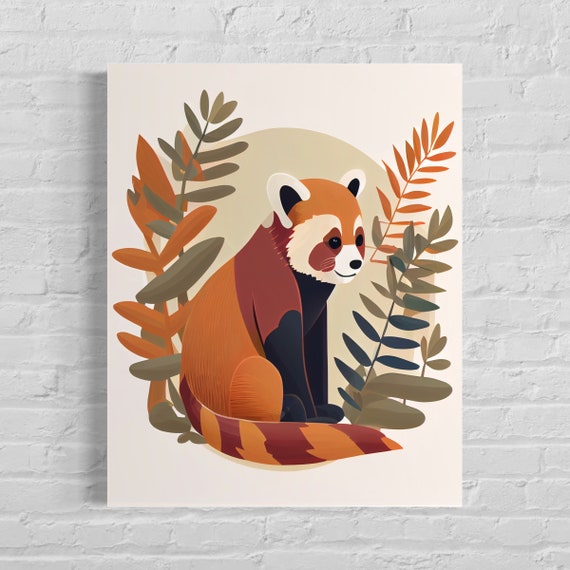Hanging on a white-painted brick wall, this artwork features an unframed, beige-toned poster showcasing a captivating illustration of a red panda. The panda, rendered in a style reminiscent of a mid-century modern aesthetic, displays vibrant fur that transitions from darker reds on the upper body to lighter oranges towards the rear end and legs. Its expressive face is highlighted by beige fur around the eyes, which are black and accented with darker red marks beneath them. The panda's ears are trimmed in beige with black insides, while its arms and paws are a stark black. The tail, which curls towards the panda’s front, is strikingly striped in alternating dark red and lighter orange hues. This charming creature stands on its hindquarters, seemingly smiling and gazing off to the left. Surrounding it, various ferns and foliage in shades of green, rust, olive, and burnt orange provide a lush background. The artwork is further characterized by a large beige circle behind the panda, possibly symbolizing the sun, adding a sense of warmth and cohesion to the serene composition.